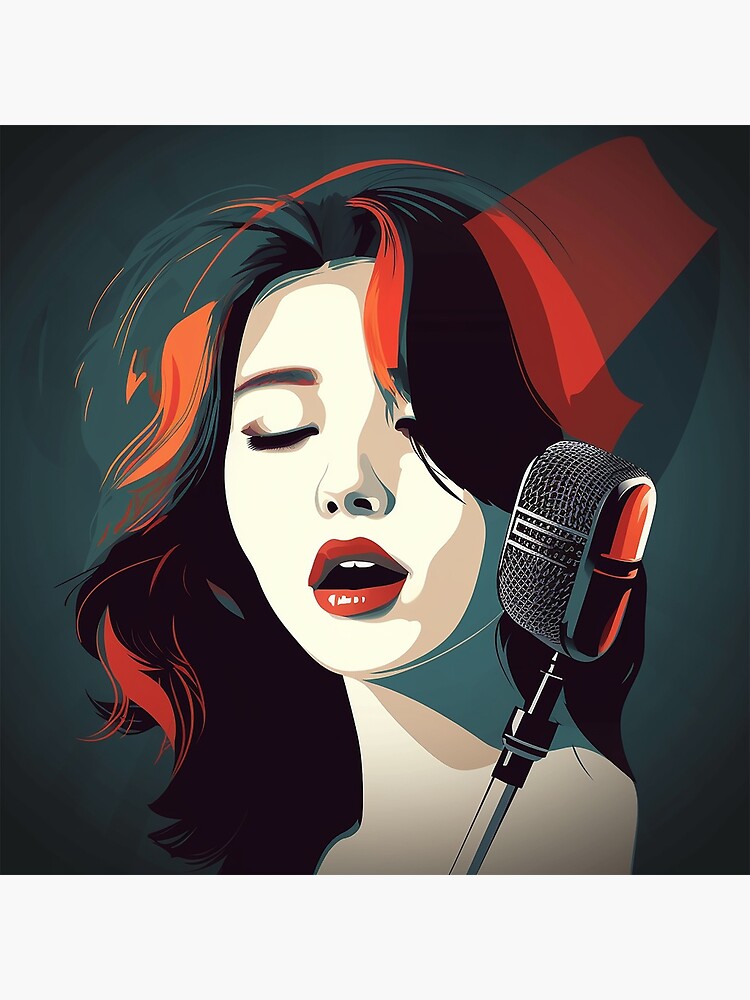The digitally created image features a woman with closed eyes, seemingly lost in thought or perhaps singing into a microphone positioned on the right side of the frame. The background is a dark teal or deep forest green. The woman has long, wavy black hair adorned with abstract layers of red, orange, and turquoise that catch the light. Her face, with its pale ivory or cream complexion, showcases bright red lipstick and a glimpse of her top teeth. Her visible eye and eyebrow are partly obscured by her vivid hair, and delicate shadows are cast across her face. The microphone next to her displays a reflection of the surrounding abstract colors. The overall impression is that the woman is a music artist, absorbed in her performance.